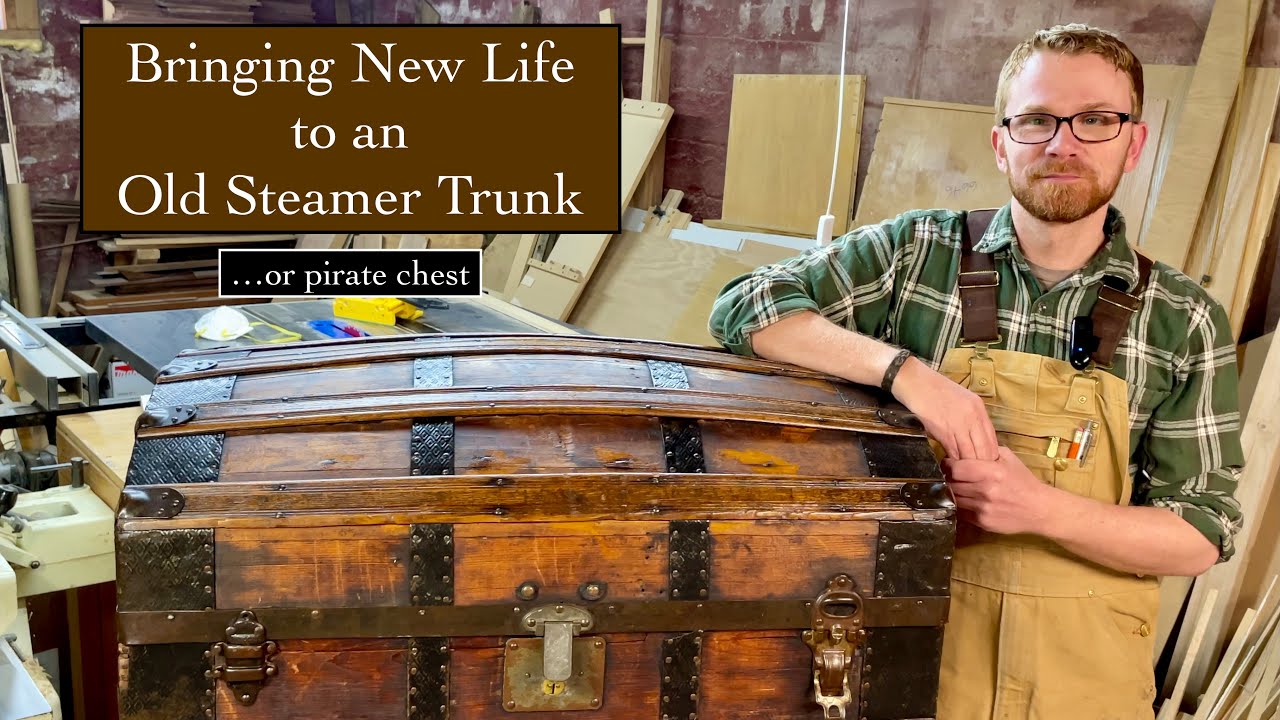In the image, a colour photograph in landscape orientation, a man stands beside a large, vintage chest in a workshop. The man is dressed in light brown dungarees with dark brown shoulder straps and a green-and-white checkered shirt. He has a light brown beard and moustache, short hair, and wears thin-rimmed black glasses. A leather bracelet is visible on his right hand, which is resting on the chest, while his left hand lightly holds his right fingers. 

The chest, resembling a treasure chest, is the focal point in the foreground, characterized by leather straps running from back to front and wooden straps running left to right. It features three metal clasps on the front—a bronzy clasp on the left and right, and an aged, slightly rusty one in the middle.

On the top left of the image, there are two text boxes. The larger brown rectangle with a thin black outline reads, "Bringing new life to an old steamer trunk," while a smaller rectangle below it, with white text over a black background and outlined in white pencil, says "...or pirate chest."

The background reveals a workshop, with various light beige wooden panels leaning against a reddish-brown wall. A workbench cluttered with items, including what appears to be a white face mask, lies behind the man on the left-hand side of the image. A vice is attached to the left side of the bench. The entire scene suggests that the man may be a furniture refinisher showcasing his work on the chest, possibly for his website or channel.